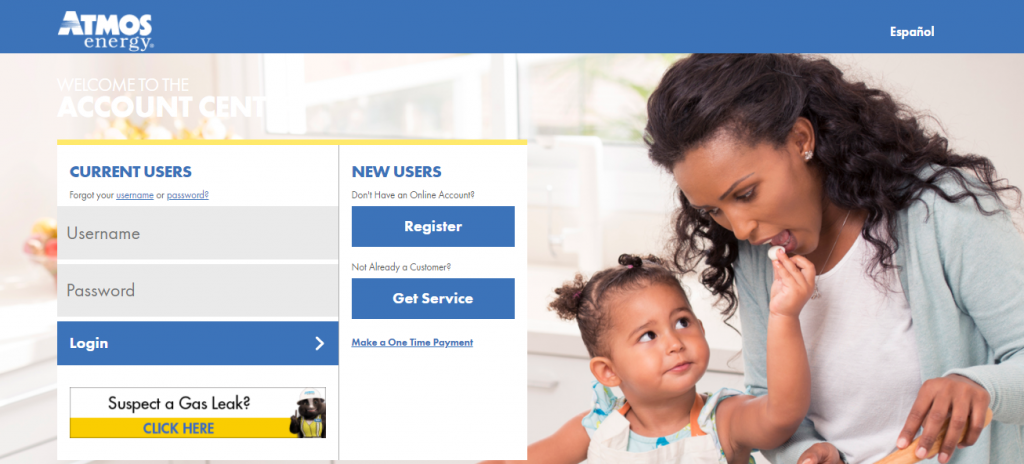This image is an advertisement for Atmos Energy. The top section features a blue banner that runs the entire width of the image, with "Atmos Energy" prominently displayed. On the far right of this banner is the word "Español."

The background sets a warm and homely scene within a kitchen. In the foreground, a woman dressed in a white top and a lime green cardigan is slightly bent over a countertop, apparently in the midst of baking, possibly making cookies. Adjacent to her, a little girl dressed in a multicolored dress featuring shades of orange, teal, and white, with her hair styled in tiny pigtails, is playfully trying to feed the woman what appears to be a small white treat, perhaps a marshmallow.

On the left side of the image, there is a prominent box for Current Users, containing fields for username and password, an option for those who forgot their username or password, and a blue "Login" button. Below this section, there is a New Users area which offers options for those who do not yet have an online account to register, and for those who are not already customers to get service. Additionally, it provides an option to make a one-time payment. A crucial safety feature is also included in this section: a yellow "Click Here" prompt for users to report if they suspect a gas leak.